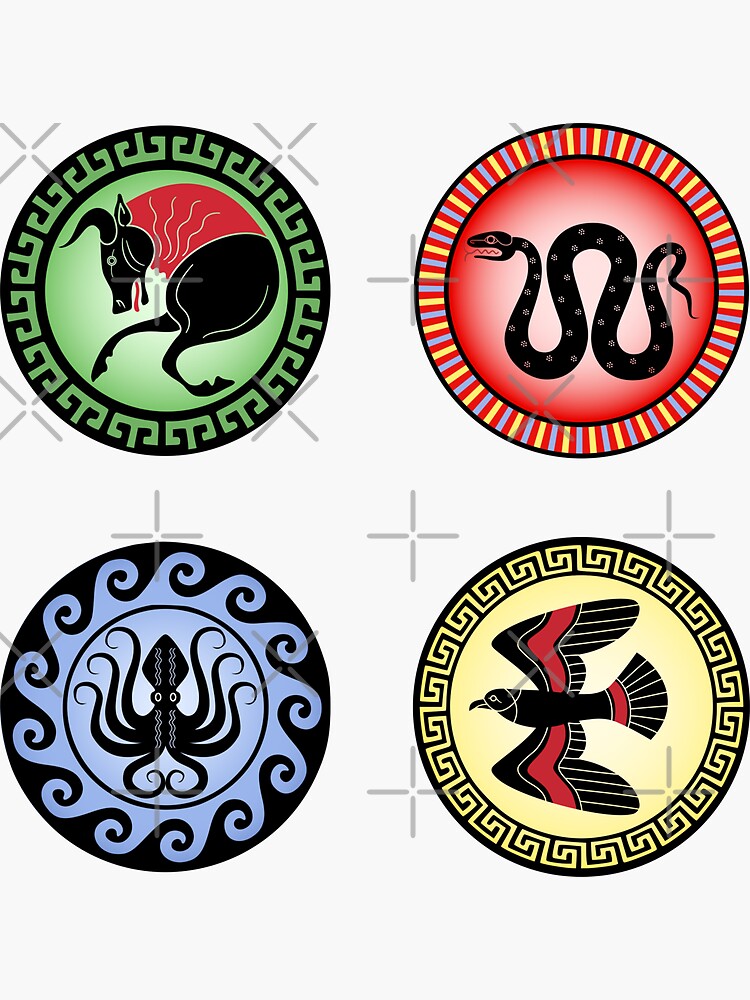The image features a white background adorned with an alternating pattern of x's and plus signs. The top row displays three x's, followed by a row of three plus signs offset slightly to the right. This alternating pattern of x's and plus signs continues vertically with three rows of each. 

Superimposed on this background are four distinct, circular images, each with a different animal at its center. 

1. The top left circle is green with black designs around the edges, showcasing a red-maned horse or bull with only its front legs visible and holding a red cape.
2. The top right circle is predominantly red, bordered by rainbow colors, and centers on a black squiggly snake.
3. The bottom left circle features a blue background with wave-like designs and a black octopus or squid in its center.
4. The bottom right circle is yellow and contains a black bird in flight facing left, adorned with red stripes on its wings and tail.

Each circular image adds a distinct splash of color and thematic variation to the geometrically patterned background, suggesting symbolic representations of various animals.